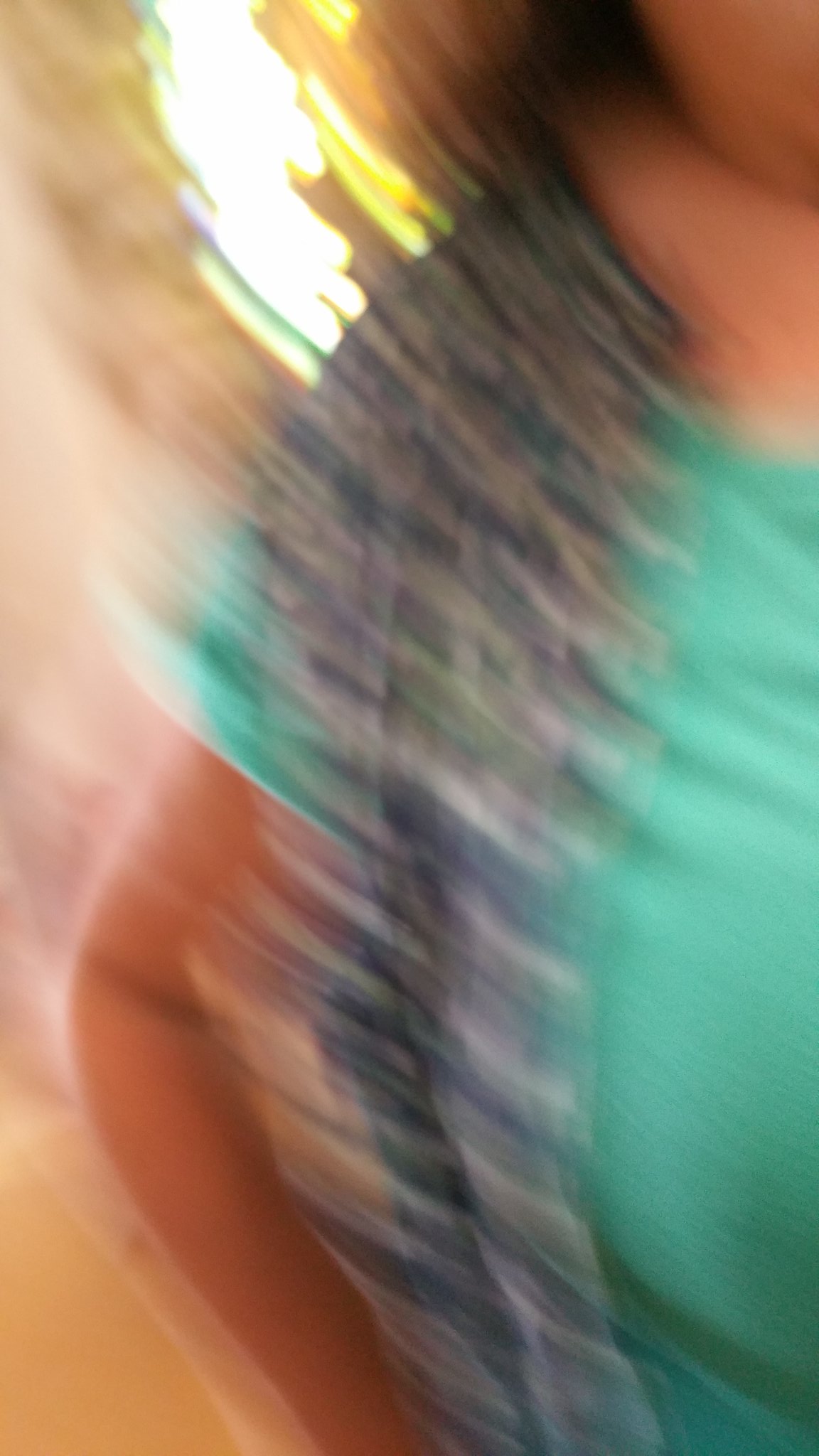The image features a young child with their face obscured, creating ambiguity about their identity. The child, potentially a little girl, is dressed in an aqua teal-colored short-sleeve shirt, which appears to be layered with some type of vest. Visible details include the child's arm, part of the chest, chin, and a bit of hair. Adding to the complexity, there's a blue and white striped object draped over the child's arm, though it's difficult to discern exactly what it is due to the overall blurriness of the photograph. The background is completely blurred as well, with an indistinct light source contributing to the obscure and dreamy quality of the image.